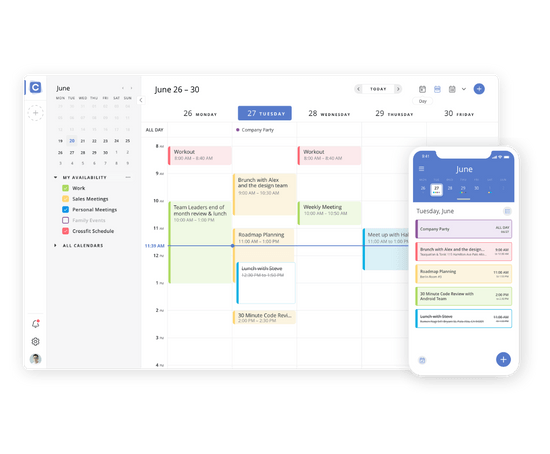The image is a detailed screenshot of a calendar application, showcasing a user interface with multiple components. The main focus of the screenshot is a horizontal rectangular calendar display that features a pop-up window resembling the size and shape of a cellphone screen, which highlights specific appointment details for a selected date.

In the upper left-hand corner of the image is an icon of a blue square containing a white "C," signifying the app's logo. The majority of the page is white, except for a grey strip on the left-hand side, which includes a miniature calendar for the month of June. In this mini-calendar, past dates are greyed out while the current and future dates are displayed in black, starting from Sunday, June 19, and extending into early July.

Below the mini-calendar, there are categorized listings of different types of appointments. The main area of the page emphasizes the week of June 26-30, with a clear highlight from Monday, June 29, through Friday, June 30. Particularly, Tuesday, June 29, is highlighted in blue, indicating its significance or selection. The inset window showcases several detailed appointments and events specifically for June 27.